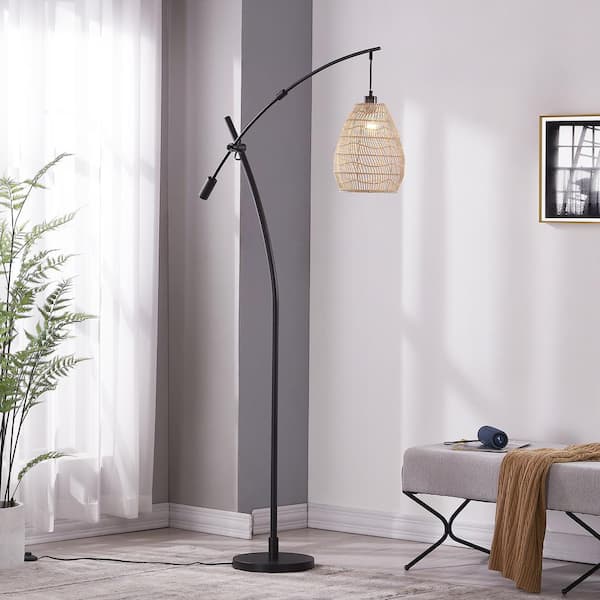The image showcases a corner of a room with light gray walls and a darker gray accent wall that features white borders at the bottom. The floor is covered in white tiles with occasional flecks of color. A large window with white curtains allows natural light to filter into the room. Positioned against the lighter gray wall is an intricately framed picture with a gold and white frame, although its detailed content remains unclear due to reflections. Beneath the picture, there is a stylish backless chair, or possibly a long stool, draped with a brown sweater.

Occupying the central space is a striking, tall floor lamp with black metal construction and a wicker basket-like shade. It features an arched top with a drop-down light that has a net over it. In the corner where the two walls meet, there's a tall, leafy green plant housed in a white ceramic pot, adding a touch of nature to the otherwise modern decor. This thoughtfully arranged interior combines elegance with understated simplicity.